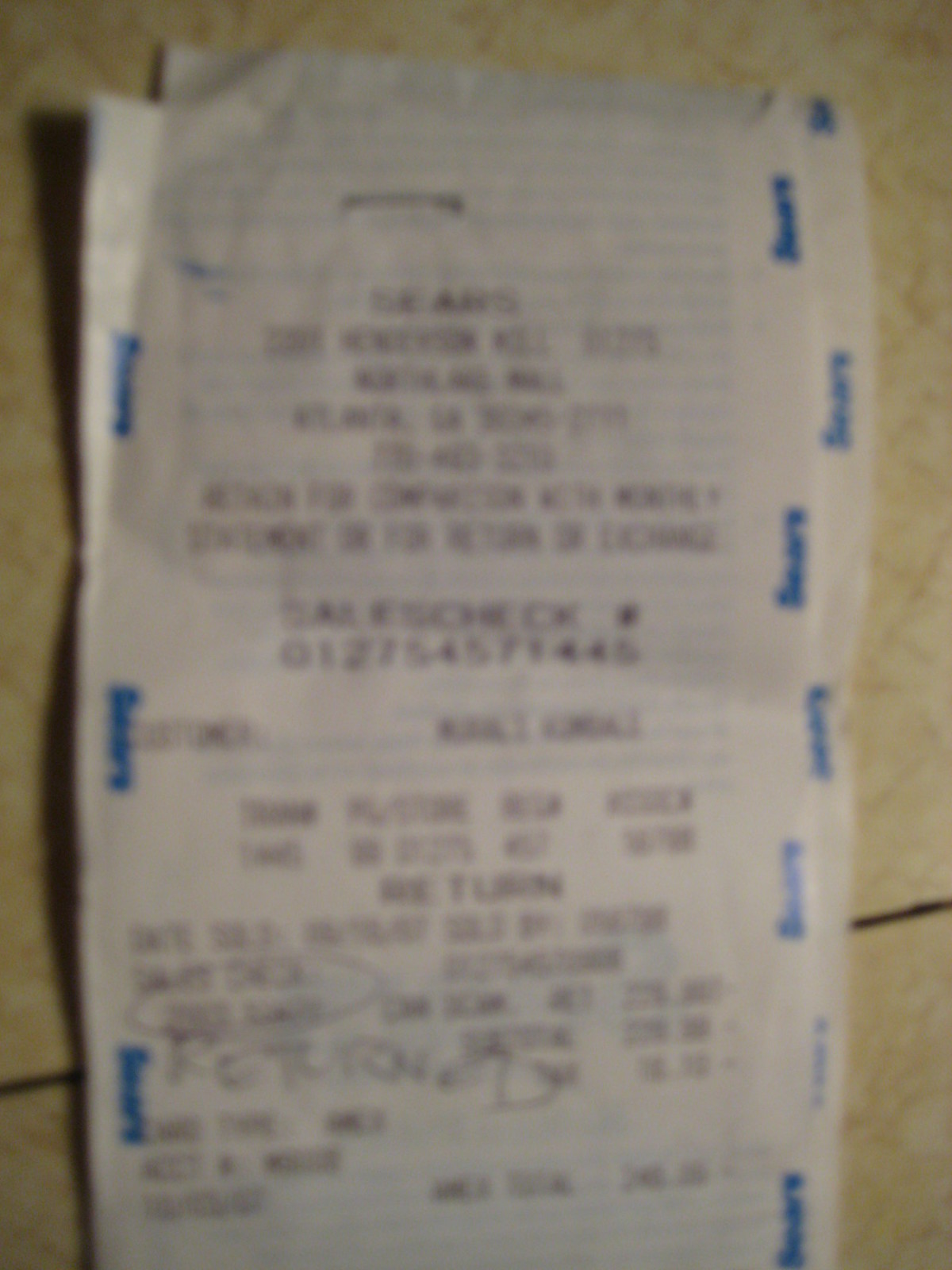In this image, we see two identical receipts laying on a tiled floor. The receipts are white, with blue writing running down their sides. The printing on the back of each receipt is prominently bleeding through onto the front, making the text somewhat difficult to read. Although the receipts are quite long, the specific items purchased are indiscernible. Each receipt does display a "SALE CHECK NUMBER" followed by a lengthy numerical sequence. The top portions of both receipts are also obscured, preventing the identification of the store from which they originated. The floor beneath the receipts consists of tan and cream-colored tiles, arranged in a grid pattern and interspersed with brown grout lines.